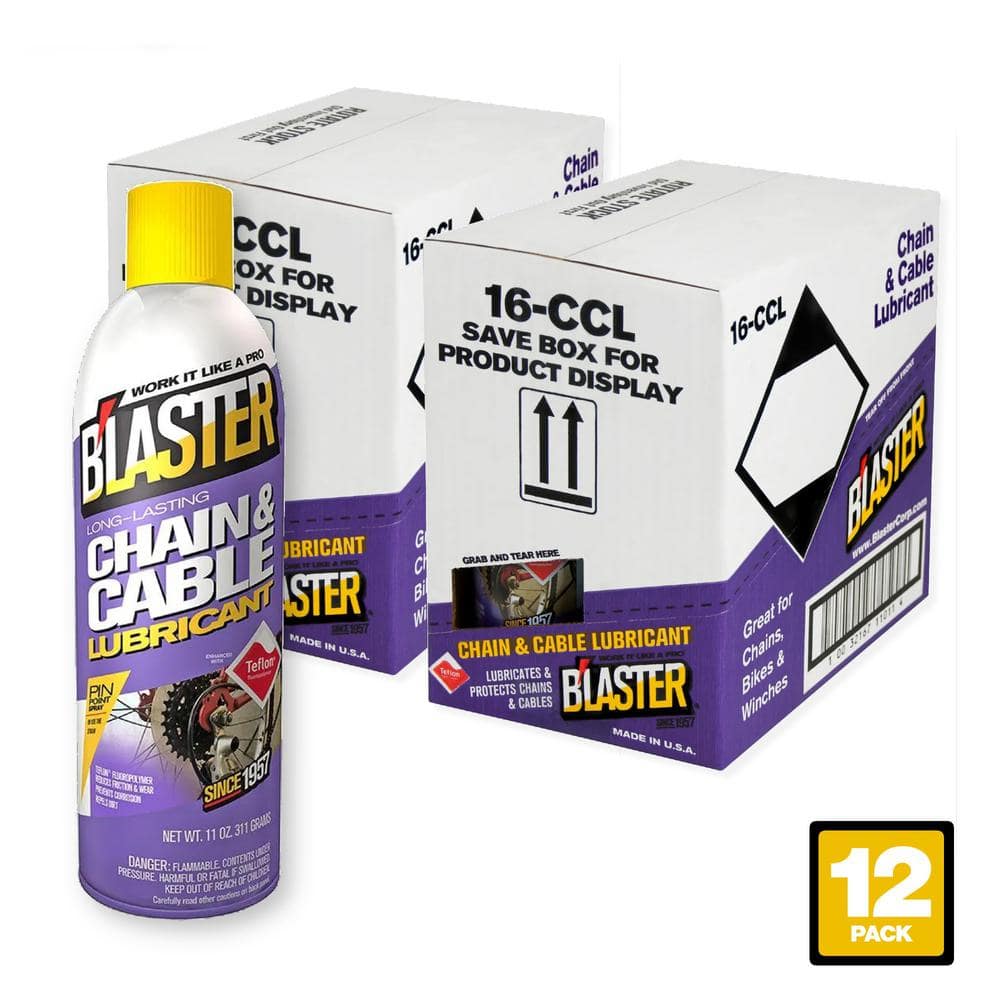This is a detailed photograph resembling a product advertisement for Blaster Chain and Cable Lubricant. The primary focus is on a spray bottle prominently displayed on the left side. The bottle features a purple and white gradient design with a yellow cap. The label, adorned with a black background split into white and yellow sections, reads "Blaster" and "Long-Lasting Chain and Cable Lubricant," accompanied by the tagline "Works like a pro." The label also includes a small image of bicycle spokes, highlighting its application for bicycle chains, among other uses. The product specifications note a net weight of 11 ounces and the text "Since 1957."

In the background, two cardboard boxes containing the same product are visible, sharing the purple and white color scheme with additional black, yellow, and red accents. One of these boxes displays the text "16 CCL, save box for product display" along with a barcode and mentions its suitability for chains, bikes, and winches. Both boxes prominently feature the product name. In the bottom right corner of the image, there is a yellow square with white text indicating a "12-pack." The overall design and layout effectively emphasize the product's branding and versatile use.